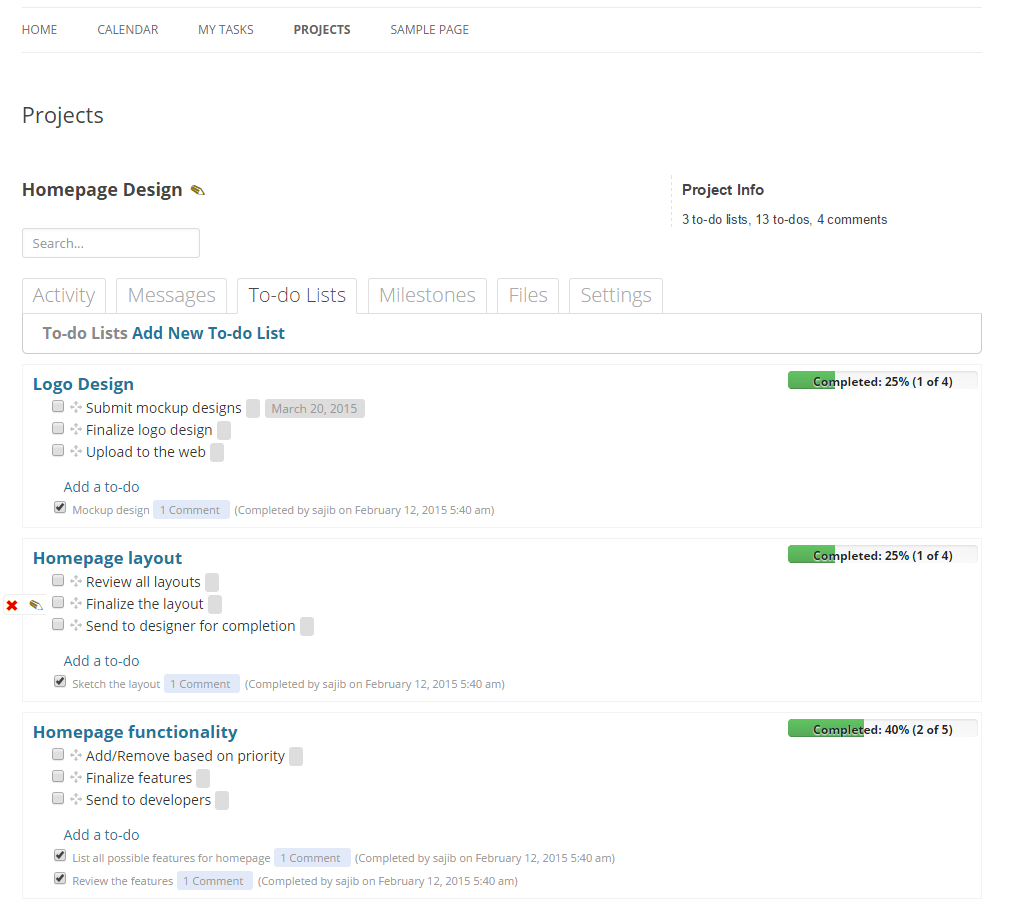The image depicts a digital project management interface with a clean, minimalistic design. 

The background is predominantly white, accentuated with thin gray lines. At the top, there's a section labeled "home calendar, my test" in dark gray text, followed by "projects" in bold, with "same page" in regular gray text distributed over thin gray lines.

Below this heading, a spaced section starts with the word "projects" in black, followed by "home page design" also in black. Adjacent to this, there's a search box outlined with a grayscale border, containing the placeholder text "search…".

Further down, in black text, the section "project info" provides details: three to-do lists, 13 to-dos, and four comments. Below that, multiple tabs span across the top of a secondary interface. The tabs' background is white, with their names in light gray text: "activity," "messages" (highlighted in a slightly darker gray since it's the active tab), "to-do lists" (also slightly darker), "milestones," "files," and "settings."

The "to-do list" tab displays various tasks. "Add new to-do list" is prominently displayed in gray text within this section. 

Underneath, a task list includes:
- "Logo design," with a sub-task "submit mock-up designs" due March 20th, 2015, further instructions to "finalize logo design" and "upload to the web." A blue "add to-do" button is present, and a task with one comment indicates "25% completed (1 out of 4)."
- The "home page layout" section, marked in light blue, contains sub-tasks: "review all layouts," "finalize the layout" (which has a red X indicating it's a critical task), "send to designer for completion." Again, a blue "add to-do" button accompanies this, showing "25% completed (1 out of 4)."

Overall, the interface visually organizes project management tasks efficiently, separates sections using a minimalist design, and uses color to distinguish between various elements and their statuses.